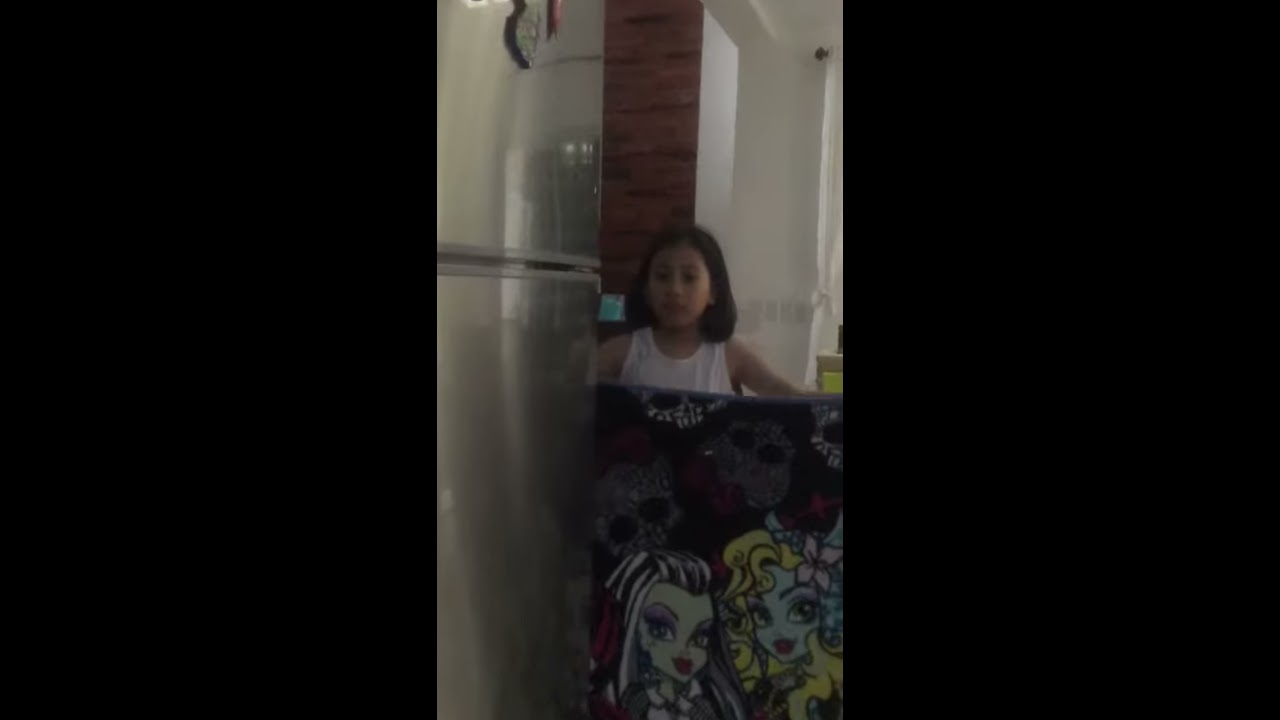The photograph features a young girl, approximately 10 years old, standing in a kitchen beside a grey, double-door refrigerator adorned with a couple of stickers on its top half. The kitchen features a white wall in the background and a segment of a wall with a gold and wooden design. The girl has shoulder-length brown hair and is wearing a white, sleeveless top. She holds up what appears to be a blanket or towel, featuring unique cartoon characters; one has yellow hair with mint green skin and a pink flower clipped on the side of her head, while the other has pink hair with light green skin. There is also a small skeleton image and another character with violet hair and eyes, and dark red lipstick. The overall image is somewhat underexposed and might have been taken in a mirror as the girl holds her cell phone above her right shoulder. To the left of the image, a shower indicates part of a bathroom setting, adding to the complexity of the scene.